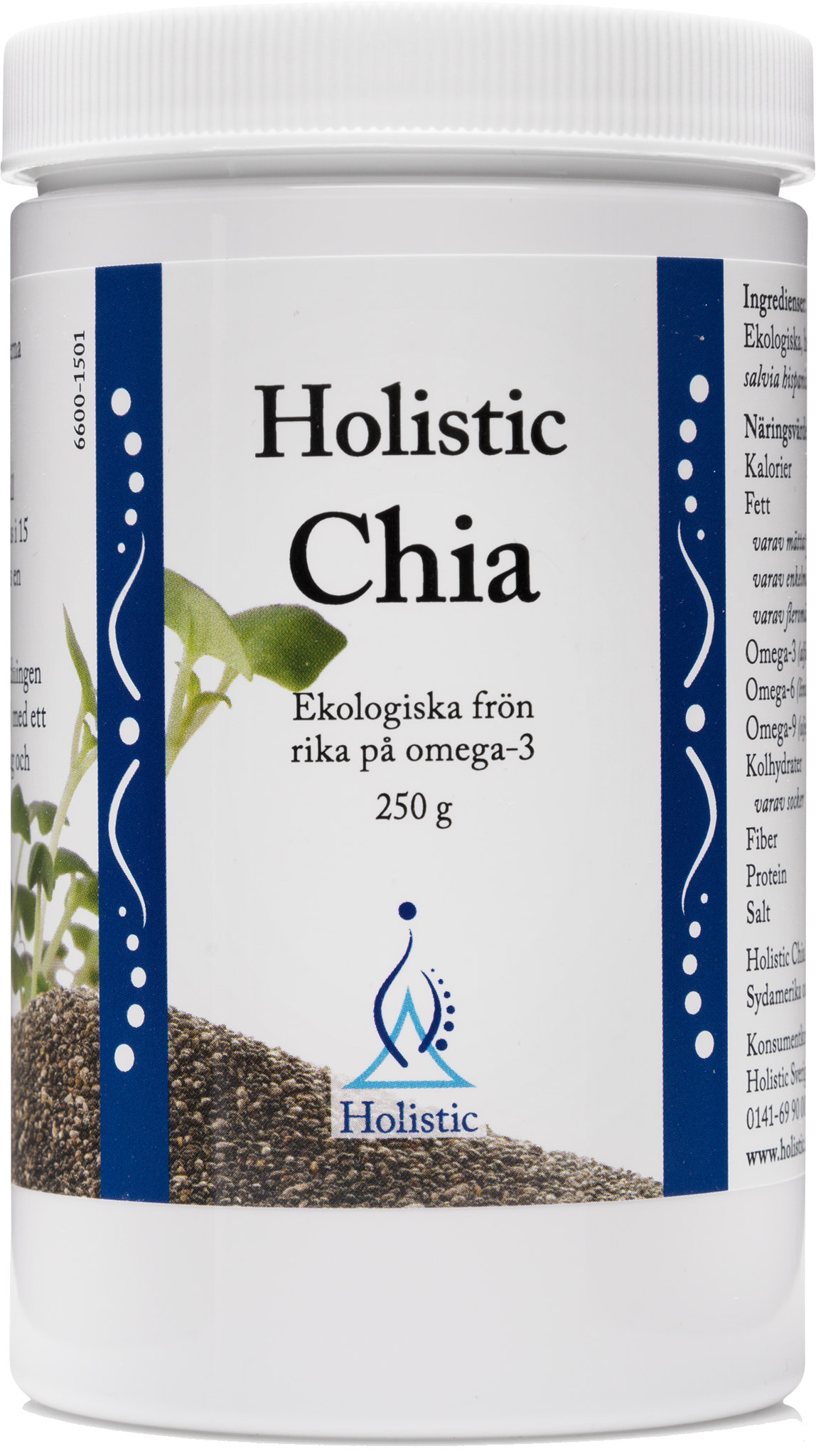This is a detailed photograph of a white plastic bottle with a screw-on lid, containing Holistic Chia seeds. The bottle is set against a plain white background. The label on the bottle is prominently designed in black and various shades of blue, featuring the text "Holistic CHIA" at the top, followed by two lines of text likely in a Scandinavian language (E-K-O-L-I-G-I-S-K, E-K-O-L-O-G-I-S-K-A, F-R-O-N). Below this text, "250 grams" is clearly marked. A logo composed of a triangle and two curves with the word "Holistic" written underneath separates the top text from additional details below. The label also incorporates illustrations of green chia leaves and seeds, emphasizing the organic and nutritional aspect of the product. Flanking the central text are two blue vertical banners adorned with white dots and squiggles, running the length of the bottle. These banners contribute to the label's decorative appeal. Some numbers and additional product information are present but partially cut off by the photo, making them indistinct. The overall design exudes a clean, holistic aesthetic, indicating a health-focused product.